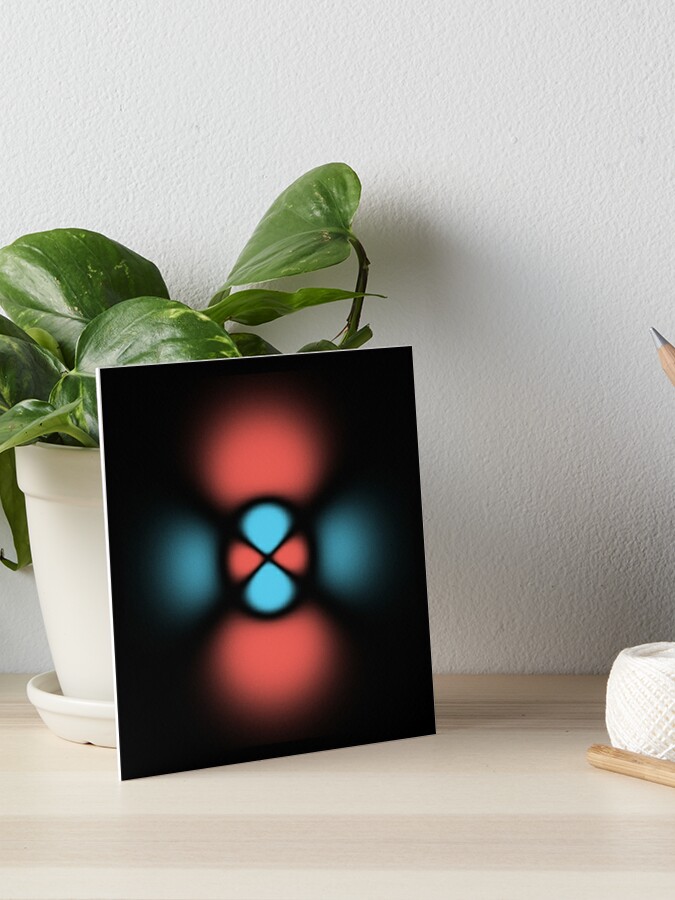The image features a vibrant, abstract design set against a black background. The design consists of two large red spheres positioned at the top and bottom, with smaller blue spheres flanking the left and right sides. At the center, additional blue shapes are arranged vertically while red shapes sit horizontally. This intricate design is placed adjacent to a lush potted plant, which has broad, green leaves. The plant is contained in a white pot that rests on a matching white tray. The background boasts a pristine white wall, and the ensemble is all set atop an off-white table. To the right of the main focus, there appears to be another white pot, possibly containing some wooden elements, although its exact composition is unclear.